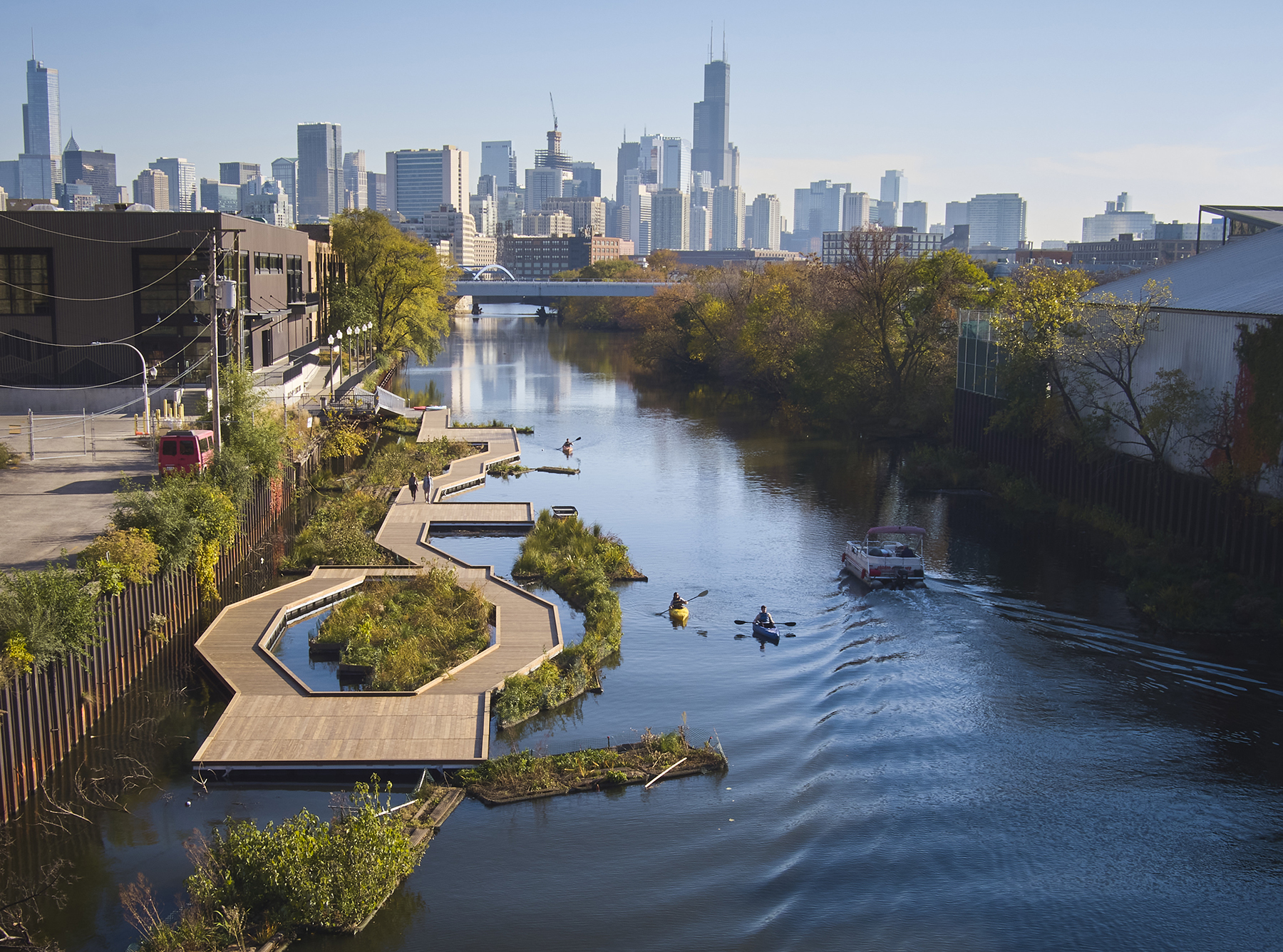The image depicts a vibrant outdoor scene featuring a river that flows from the foreground into the distance. In the lower right, a small white rectangular boat, creating a visible wake, adds dynamic movement to the dark brown-blue waters. Two kayakers, paddling towards the camera, enhance the sense of activity.

To the right of the river, lush green trees line the banks, extending towards a whitish warehouse-like building. On the opposite side, a complexly shaped dock, with hexagonal or multi-sided sections, juts into the water. This area is surrounded by growing green grass and leads to a paved, winding walkway, some parts of which seem to float over the water. Adjacent to this intricate dock is a large brown warehouse building.

In the background, a bridge spans the width of the river, stretching towards a distant city skyline characterized by towering skyscrapers. Above, the sky is a light blue with scattered white clouds, contributing to the bright and clear atmosphere of the scene. The overall clarity of the image highlights the distinct elements and vibrant details of this lively waterside urban landscape.